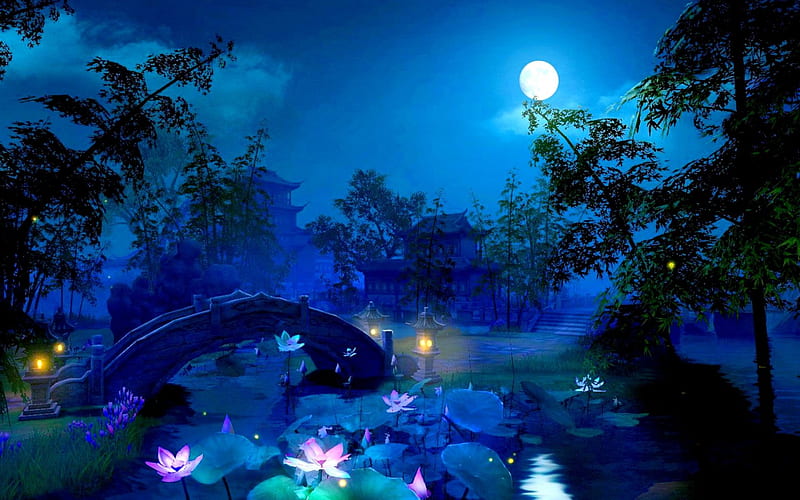This image is a detailed, illuminated painting, seemingly computer-generated, portraying an enchanting landscape with a strong blue hue. At the center of the scene, a serene body of water, possibly a river or pond, is adorned with blooming pink lotus flowers and lily pads. The water body is crossed by a small, stone arched bridge, which connects the left and right banks. On the right shore, a pathway extends from the bridge, leading to a stairway that ascends toward two large, Chinese-style buildings with gracefully upturned eaves. The buildings, surrounded by tall, lush trees and verdant grass, blend seamlessly into the picturesque landscape. The trees lean in various surreal angles towards the water, enhancing the ethereal atmosphere of the scene. Illuminated lamps punctuate the ends of the bridge, casting a gentle glow. Above, the sky is a soft blue, dotted with white clouds and mist, and is crowned by a radiant full moon, adding a mystical quality to the entire composition.